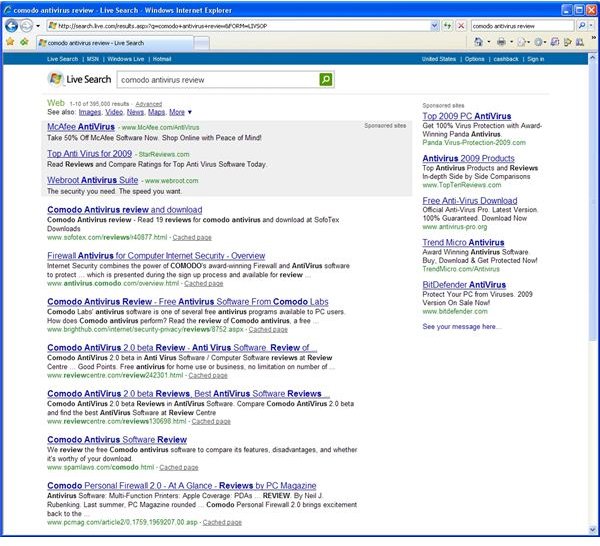This image is a screenshot of a web browser displaying a search for antivirus software reviews. The browser appears to be an older version of Internet Explorer, likely from the Windows XP era. At the top, the browser indicates the page title as "Antivirus Review" and shows "Live Search" in the search bar. Only one tab is open, which contains the search results for "Comodo Antivirus Review."

The search results page features a long list of links to various antivirus reviews, with Comodo prominently mentioned. On the right side, there is a column dedicated to sponsored sites. The interface of the browser is characterized by its dated appearance, with an all-white background and the classic Windows logo situated in the top-left corner, reinforcing the impression that this is an old Windows operating system.

The overall aesthetic is a clear throwback to the early 2000s, providing a nostalgic glimpse into past technology and internet browsing experiences.